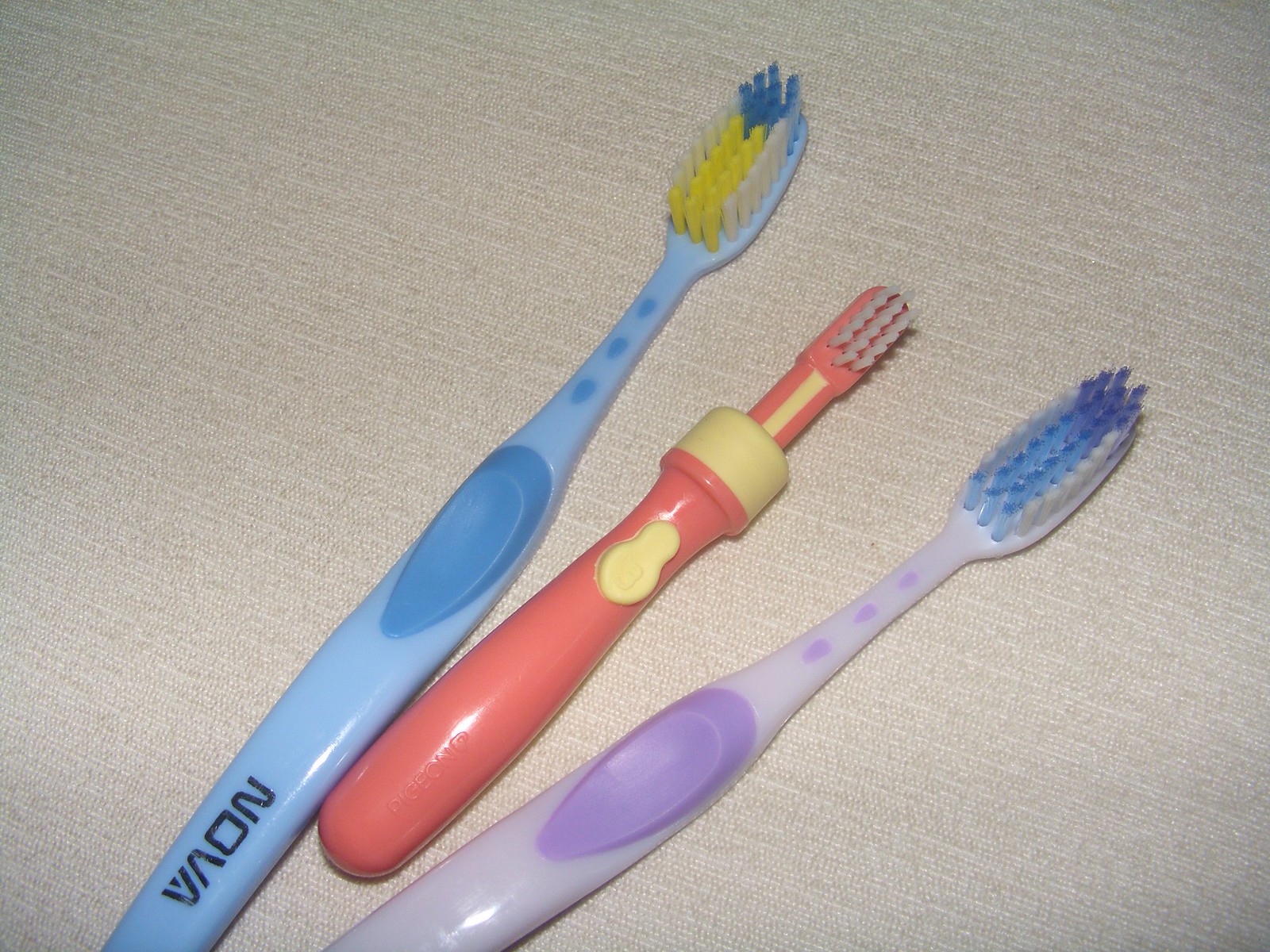The image features three children's toothbrushes arranged diagonally on a tan, almost mesh-like fabric, with the bases of the toothbrushes positioned in the bottom left corner and their heads angled toward the top right corner. The leftmost toothbrush has a blue body with dark blue highlights and a thumb handle. Its bristles are an arrangement of blue at the top, white on the sides, and a yellow section integrated in between. It also features a logo that says "Nova". The middle toothbrush, noticeably smaller and designed for a child, has a thick pink handle with a yellow spot for thumb placement, and it is equipped with small, white bristles. The rightmost toothbrush showcases a light purple body with darker purple accents and a thumb handle. Its bristles include a blue center flanked by white sides.